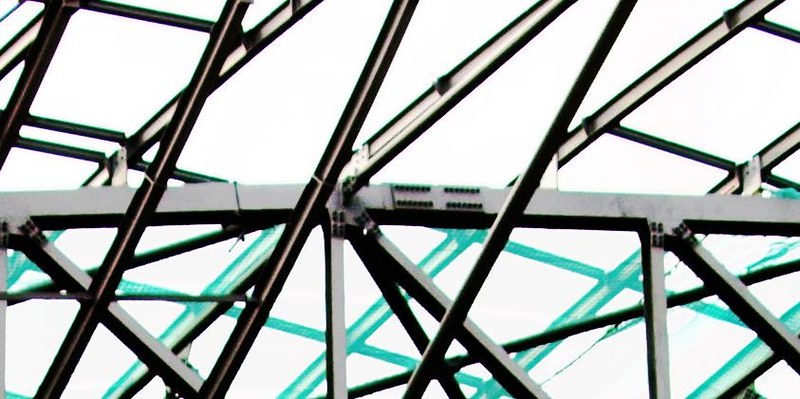The image depicts an intricate arrangement of steel beams that potentially form the upper structure of a bridge, though it might also be the framework of a steel-constructed building. The scene is viewed from below, emphasizing the geometric pattern and varied orientation of the beams. Prominent in the composition are four beams slanting diagonally to the right, intersected by others extending more horizontally. A substantial horizontal beam traverses the image's center, intersected by two vertical beams. A distinctive V-shaped beam structure is positioned centrally. At the top, a secondary set of beams extends upwards and horizontally, with a bar connecting them. The steel beams, predominantly gray, appear to transition to a teal-green hue towards the bottom, possibly reflecting light from a glass or skylight overhead. The overall color scheme varies between shades of black, white, gray, and light blue, suggesting a brightly lit outdoor setting, likely captured during daylight against a predominantly white sky.